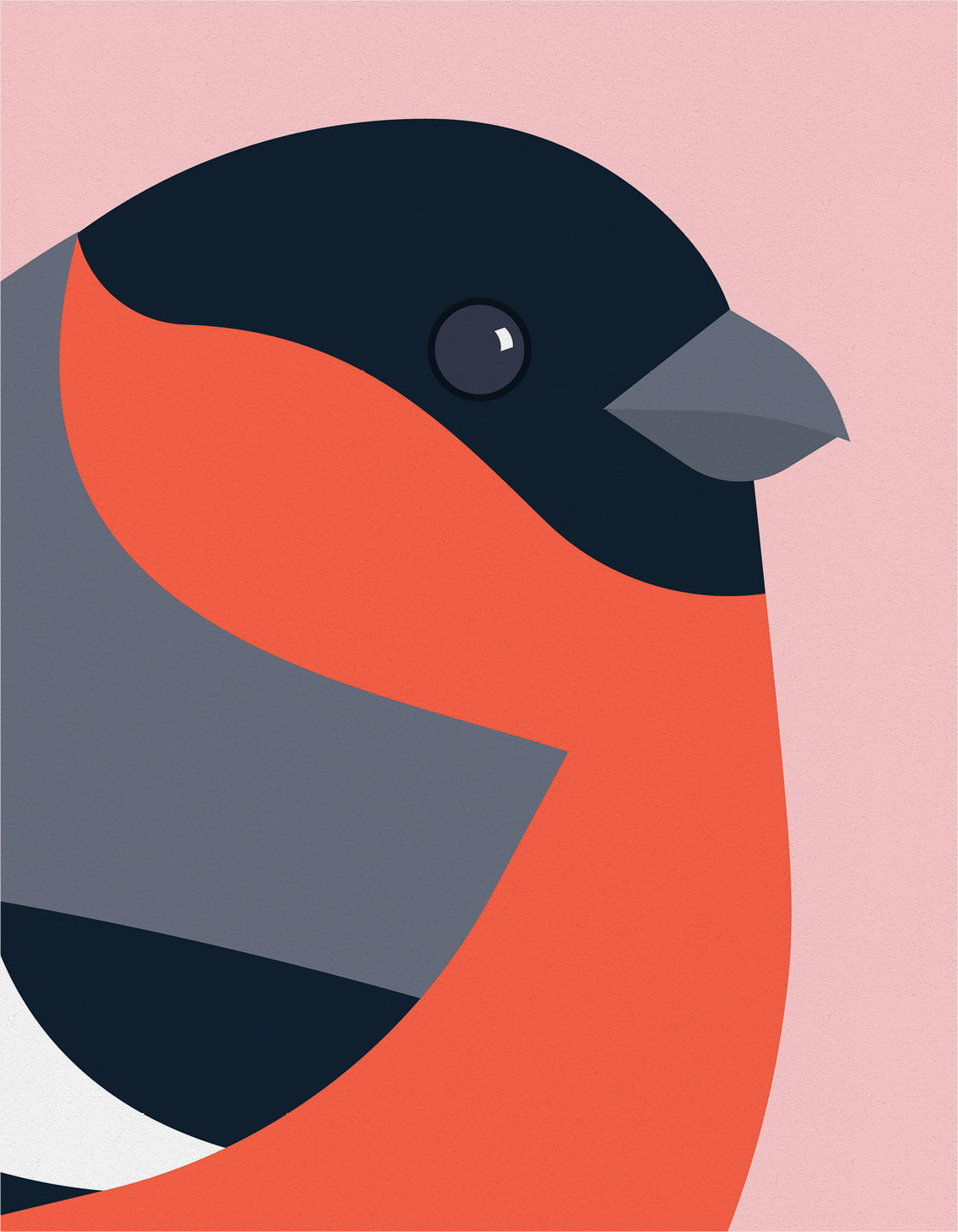This is a simplistic, stylized painting of a bird, set against a soft pink background. The bird, resembling a budgie, has a black head with a gray beak and a distinct black eye highlighted with white, outlined in black. The neck and chest are painted a bright red, while the back and shoulder area are gray. The wings show a combination of black and white. The bird has a round, almost cartoonish form, facing towards the right side of the vertical, rectangular image. The design is reminiscent of paper cutouts, with no detailed feathers, just solid color blocks indicating the bird's different parts. The bird's feet are not visible, emphasizing its simplistic and artistic aesthetic.